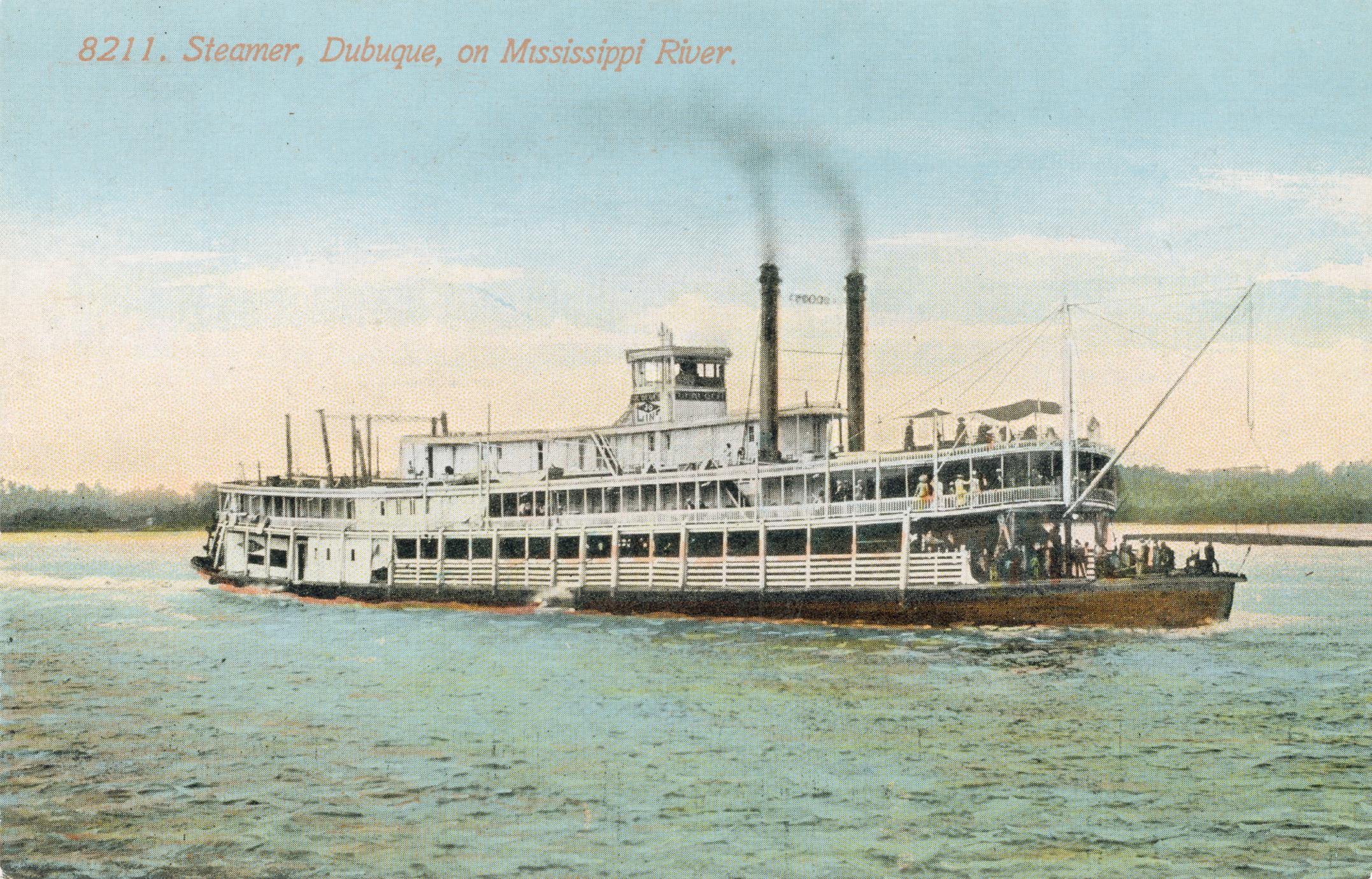This detailed vintage postcard, likely from the early 1900s, features a watercolor rendition of the "8211 Steamer Dubuque" navigating the serene waters of the Mississippi River. The steamer is prominently centered in the image, showcasing its old-fashioned, three-tiered structure. The boat's primary color is white with a deep brown or black base, emphasizing its classic design. Each level of the ship is bustling with people, the lower decks crowded, and a few individuals visible on the topmost deck. The passengers, dressed in period attire with women donning hats and dresses, add to the nostalgic atmosphere. Two steam towers release gentle plumes of smoke into the pastel-colored sky, contrasting the peaceful backdrop of the green forest and the blue-green river. The water appears still, reflecting the calmness of the scene, while support lines run to a large pole in the foreground, indicating the intricacy of the vessel's construction. This picturesque and muted landscape offers a tranquil glimpse into the bygone era of steamboat travel on the Mississippi River.